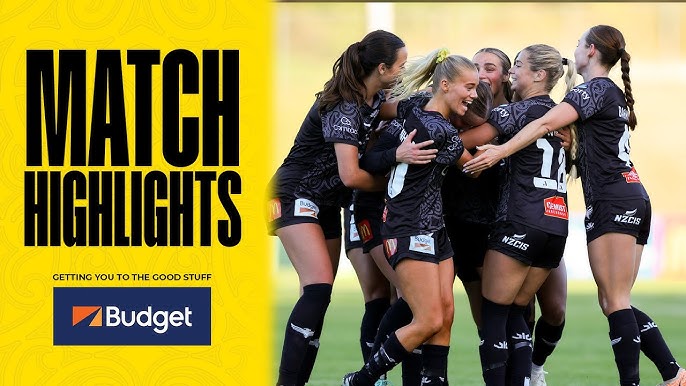This detailed magazine ad features a bright yellow background on the left third with bold black text reading "Match Highlights," followed by smaller text stating "Getting You to the Good Stuff." Below, there is a blue rectangle decorated with orange and yellow-orange triangles, containing the word "Budget" in white. The right two-thirds showcases a vividly colored image of a female soccer team in the midst of a jubilant group hug. The background is blurred, with shades of pink, green, and orange at the top, transitioning to a pale green at the bottom. The athletes, wearing black t-shirts, shorts, long black socks, shin guards, and sports shoes, have their hair tied back in ponytails or braids. Visible sponsorship logos and player numbers on their uniforms further emphasize their triumphant display, suggesting they are celebrating a recent achievement, perhaps a goal. The composition radiates happiness and unity, perfectly aligning with the ad's message of bringing viewers the highlights.